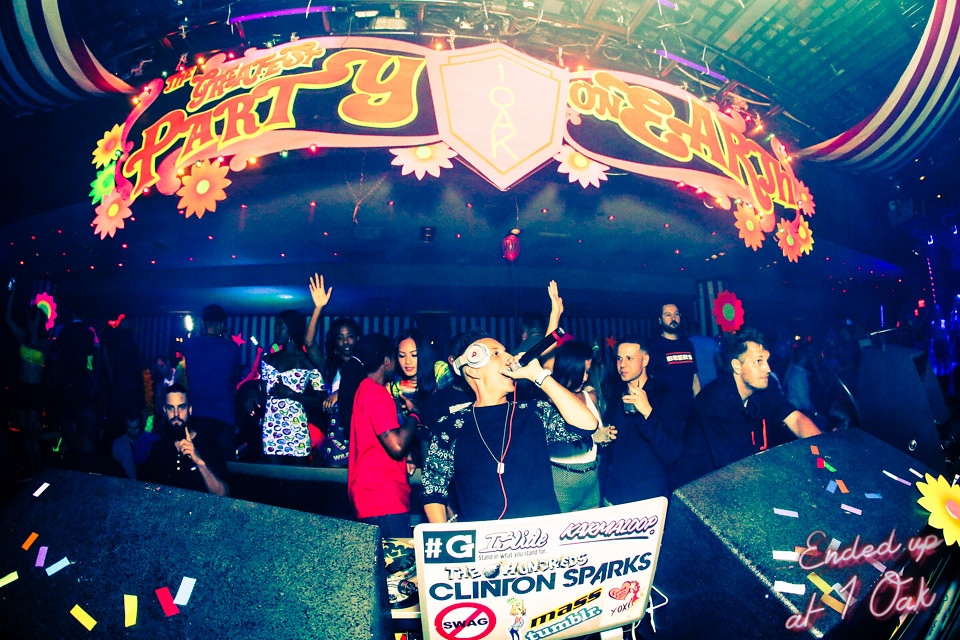This vibrant full-color photograph captures an electrifying party scene centered around a DJ holding a microphone, identified as Clinton Sparks by a white sign in front of him. The DJ, wearing headphones, engages with the crowd as he speaks into the mic. Behind him, a large, colorful banner proclaims, "The Greatest Party on Earth." The backdrop is bustling with people, some dancing and others mingling; one person in the far background waves energetically, while another, on the right, raises a finger in the number one sign. The foreground features vibrant rainbow confetti scattered about, adding to the festive atmosphere. The color palette includes shades of black, brown, red, yellow, orange, white, and various blues. Additionally, a yellow decorative fake flower can be spotted at the bottom far right corner. Text located in the bottom right corner reads, "Ended up at 1 OAK," hinting at a spontaneous and lively night out. The overall scene is captured casually, likely by another partygoer, immersing the viewer in the dynamic and celebratory environment.